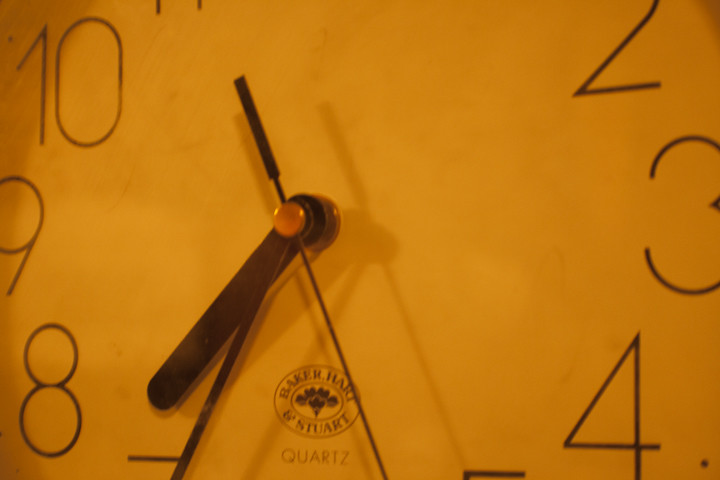A close-up image of a clock face bathed in an orange-hued filter, creating a warm, vintage ambiance. The clock’s face appears to be white, and prominently features the numbers 10, 9, and 8, with partial views of 2, 3, 4, 5, 7, and 11. The hour, minute, and second hands are clearly visible, converging around the central point of the clock. At the lower center of the clock face, a round symbol or logo from the manufacturer is noticeable, hinting at the clock's origin. The overall effect highlights the intricacy of the timepiece and evokes a sense of timelessness and nostalgia.